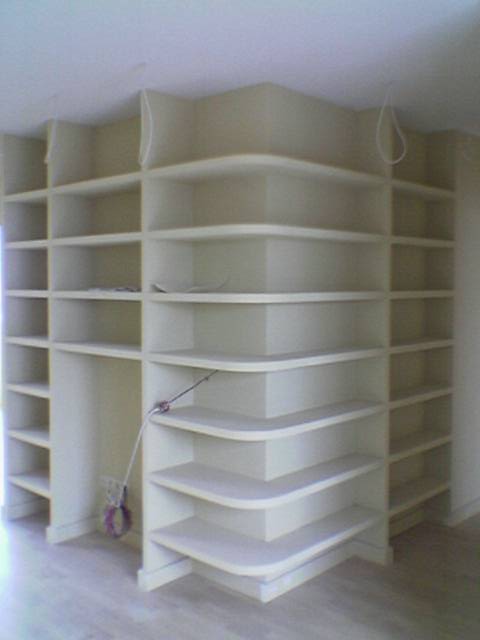This photograph features a sleek, modern corner wall installation composed of white shelving units that curve seamlessly around the corner of a room, forming an L-shape. Each shelf protrudes slightly from the wall, creating a series of open compartments that are not covered by any doors. There are seven rows of these rectangular shelves, segmented by vertical dividers into four separate sections. The wall itself has a subtle eggshell color, contrasting with the bright white shelves. Over the wall, the ceiling is an even paler white, while the floor is a smooth, light brown wood composite with a textured finish. The image, seemingly captured with an older digital camera, exhibits noticeable film grain, enhancing its vintage feel. Additionally, there are some miscellaneous objects, including a purple item with chains and some white ropes, adding complexity to the minimalist design.